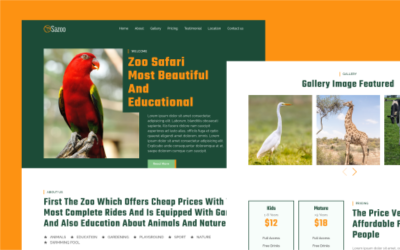Here's a cleaned-up and detailed descriptive caption for the image described: 

"The website features a distinctive orange banner at the top left, adding a vibrant touch to the page. Directly below, there's a dark hunter green rectangular section with some blurred white text at the top, making the text indistinguishable. The main navigation menu stretches from left to right across the header, though the specific menu items are also blurred.

As you scroll down, a visually appealing graphic catches the eye, displaying a picturesque outdoor scene with a clear sky and lush trees. Dominating this scene is a tropical bird, possibly a parrot, exhibiting bright red feathers and striking yellow wings. This captivating image is part of the 'Zoo Safari' theme, highlighting the zoo's status as both a beautiful and educational destination.

Beneath the graphic, there's a detailed paragraph emphasizing the zoo's affordable pricing and comprehensive rides, alongside the educational experiences it offers about animals and nature. At the bottom of the page, a small green tab on the right includes a form line for further interaction.

To the right, a white square labeled 'Gallery Image Featured' showcases images of a bird and a giraffe, inviting users to explore more of the zoo's attractions."